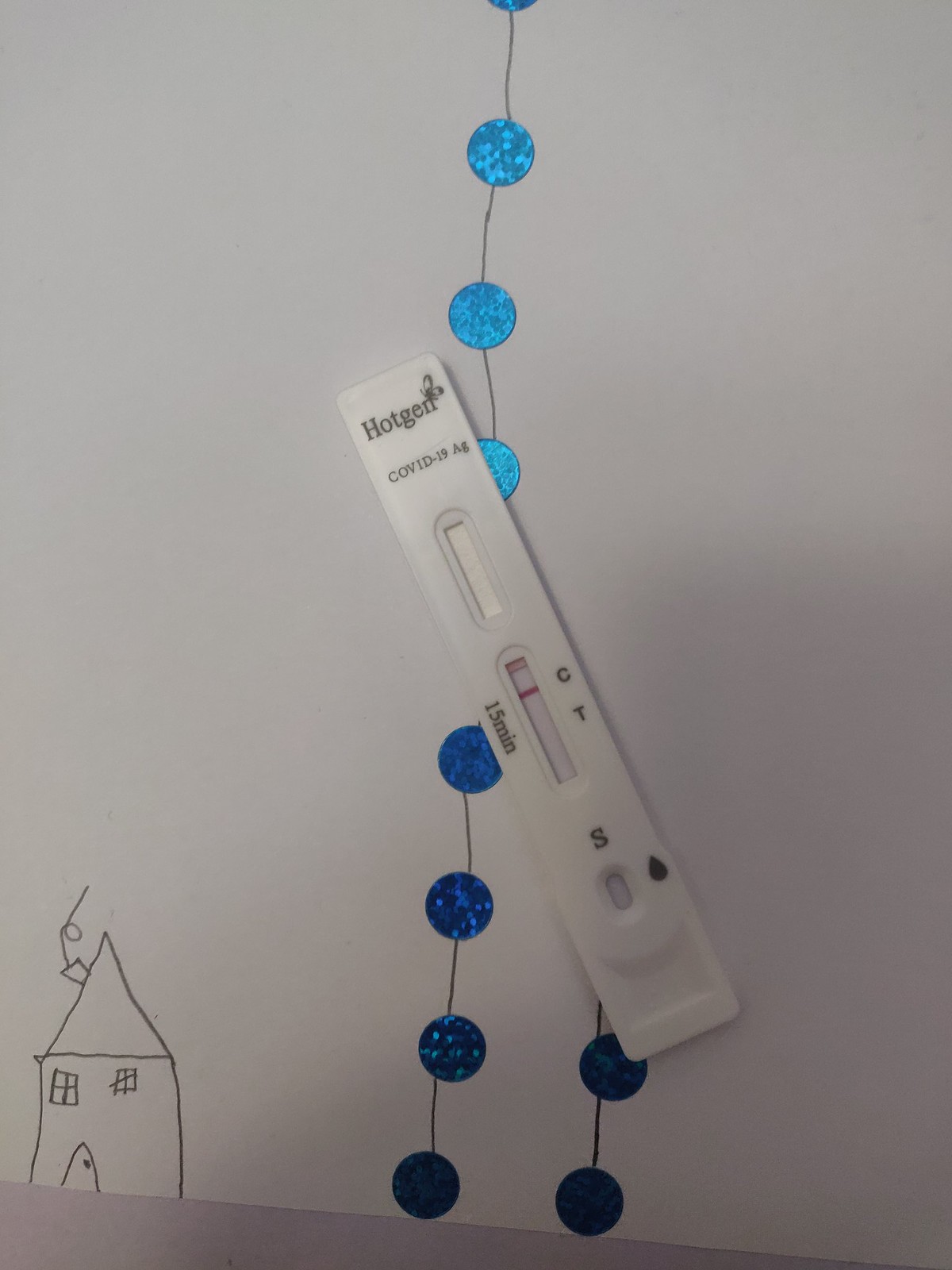The image displays a white poster board hanging against a wall, with the bottom left corner slightly slanted. The poster board features a neatly drawn illustration of a small house, complete with two windows, a door, a chimney emitting a puff of smoke, and a pointed roof. Additionally, a string or wire, which splits into two branches towards the bottom, runs vertically down the board. Attached to the string at regular intervals are round, metallic blue discs.

Atop this setting is a COVID-19 test kit labeled "HotGen COVID-19 AG." The kit specifies a 15-minute result window and includes the markers C and T, with an S window at the bottom, possibly for blood or saliva collection. One of the three windows, specifically the one labeled with a C, shows a distinct red line, suggesting it indicates the result of the test. The precise placement of the poster and test kit creates an ambiguous scene, making it unclear if they are hung on the wall or placed at an angle on a counter.